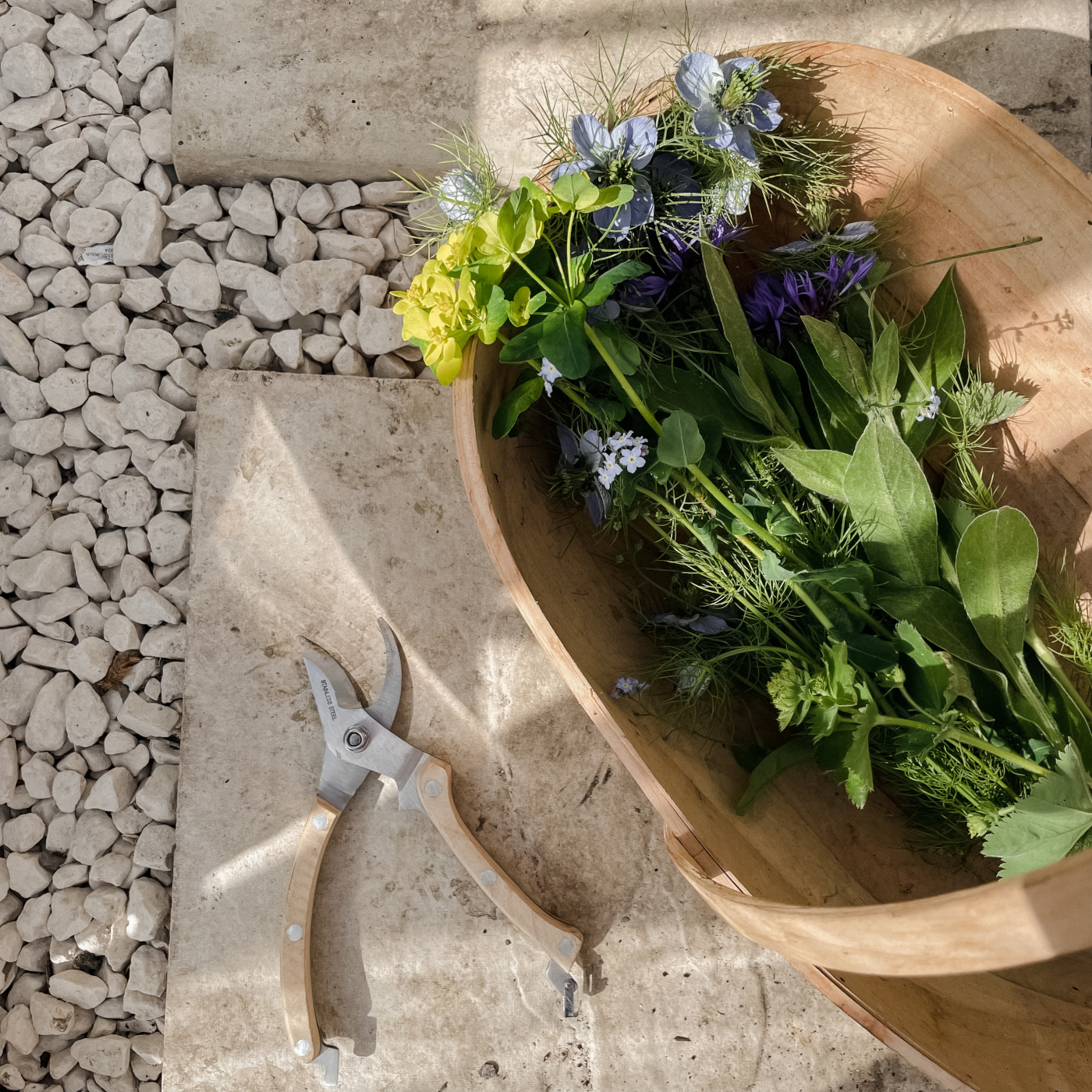The image captures an overhead view of a serene outdoor setting featuring a wooden basket filled with freshly cut flowers, set atop a stone tile. The basket, positioned on the right side of the frame, contains an array of flowers with vibrant colors—yellow, varying shades of purple, and light blues—along with their lush green stems. Notably, there are larger flowers with five petals and a few tiny lavender ones, also with five petals. To the left of the basket lies a pair of garden shears with brown handles and silver blades, placed on one of the whitish-gray stepping stones. The stone tiles are interspersed with distinctive white quartz rocks that serve as a filler, offering a textural contrast. Sunlight casts gentle shadows across the scene, enhancing the natural and peaceful ambiance.